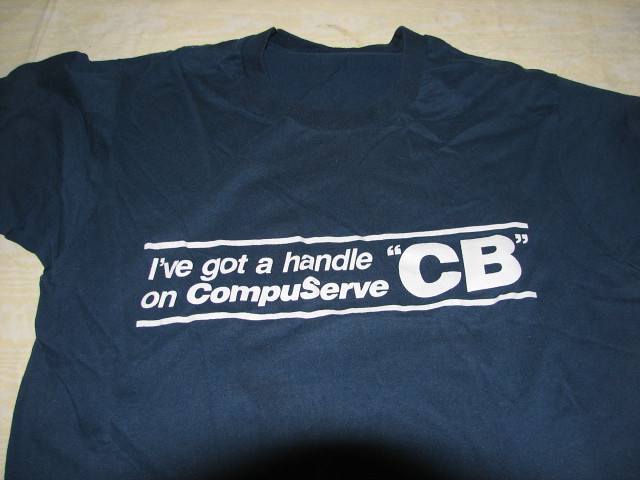The image depicts a very wrinkled navy blue short-sleeve t-shirt laid out on what appears to be a bed or a bedspread. The bedspread itself is a mix of white and yellowish hues, with a detail of a diagonal line that comes in from the top just left of the shirt, raised slightly above the rest of the cover. The shirt's collar is positioned towards the top of the picture, with its sleeves extending off both the left and right sides. Centrally, on the t-shirt, there is a graphic feature in white letters: across the top line, it says "I've got a handle," and underneath that, it reads "on CompuServe." Nearby, in larger letters, are the initials "CB" and a white line beneath them. At the bottom of the image, you can also faintly see the shadow of a person's head rounding up into the frame.